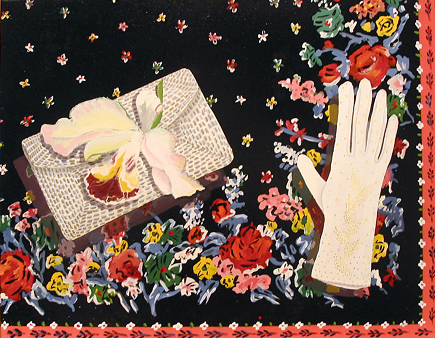The image is a meticulously crafted piece of art in a square format with a predominantly black background sprinkled with tiny flower clusters, most prominently in the top left and top middle sections. These delicate flowers come in vibrant hues of pink, yellow, and red. Central to the image is a rectangular package or handbag adorned with a flower petal that resembles a bow. This flower is white with red and yellow tips, complemented by green leaves. The right side of the image features a prominent white glove lying flat, thumb pointing toward the center, against a backdrop of larger patterned flowers. These flowers echo the colors of the smaller blooms but with greater prominence. A striking red and gold border, adorned with a leaf pattern, frames the left and right sides of the image, adding to its intricate elegance.